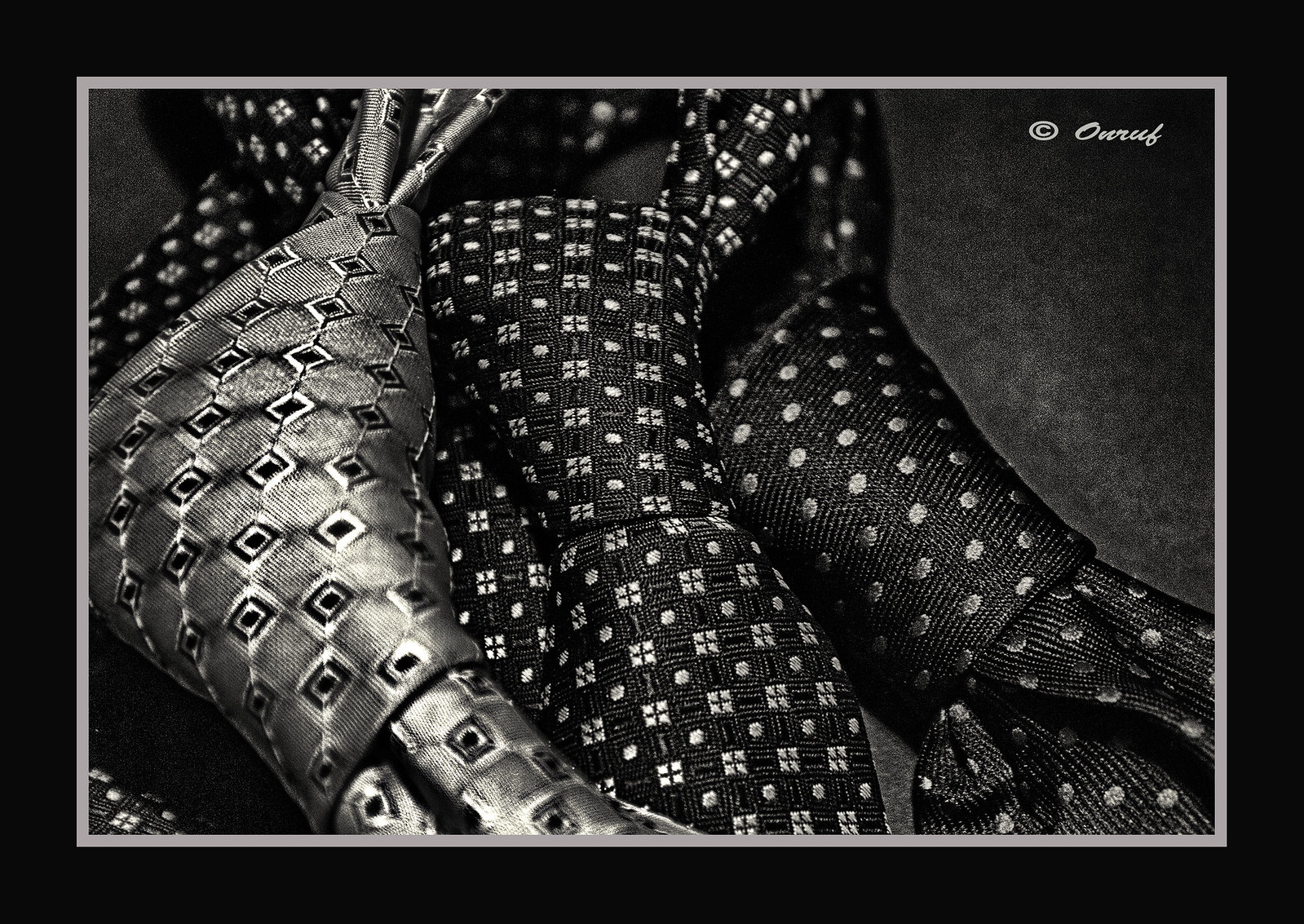This horizontally framed image features a detailed black and white realistic photograph of three neckties, prominently displayed within a thick black outer frame followed by a thin inner frame in either light gray or white. The central focus of the photograph is a close-up of the knotted section of the ties, emphasizing their intricate patterns and textures. From left to right, the first tie appears silver-gray adorned with a black box pattern, the middle tie is black featuring a combination of box and circle patterns, and the third tie on the right is black with light gray polka dots. The ties, slightly overlapping each other, create a textured, layered effect against a solid black background. In the top right corner of the image, there is a cursive signature "ANRUF" alongside a copyright symbol "©" in white text. The overall presentation is minimalist yet detailed, focusing on the refined, conservative designs of the ties.